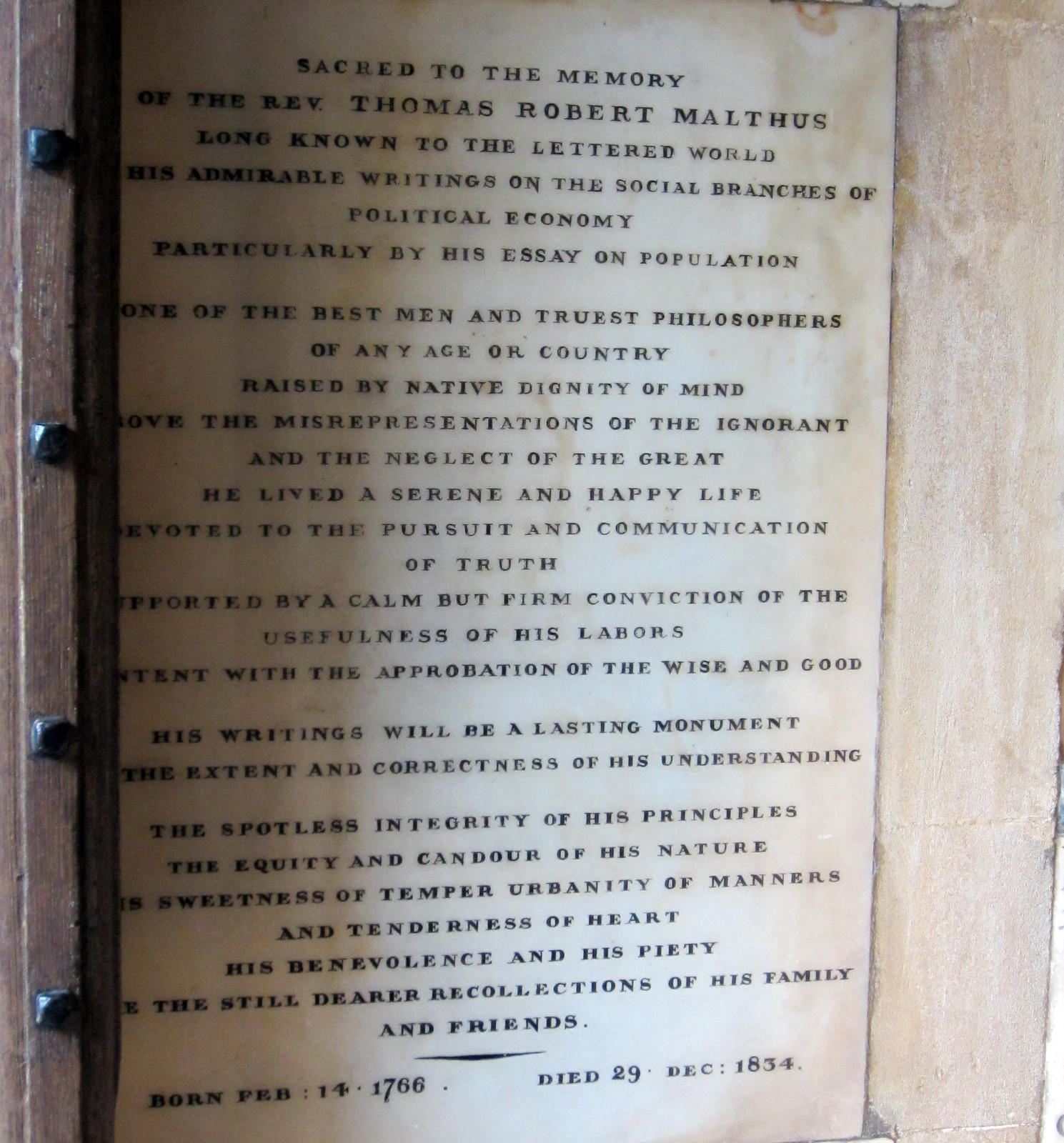This is an image of a weathered memorial plaque dedicated to the Reverend Thomas Robert Malthus, prominently positioned next to a wooden door. The plaque has aged considerably, giving it a distinguished, historical appearance. The text on the plaque, written mostly in black, begins with "Sacred to the memory of the Reverend Thomas Robert Malthus." It honors Malthus's renowned contributions to the field of political economy, particularly highlighting his essay on population. The inscription extols Malthus as "one of the best men and trusted philosophers of any age or country," praised for his serene and happy life dedicated to the pursuit and communication of truth. His writings are described as a lasting monument to both his intellectual rigor and moral integrity. The plaque states his birthdate as February 14, 1766, and his date of death as December 29, 1834.